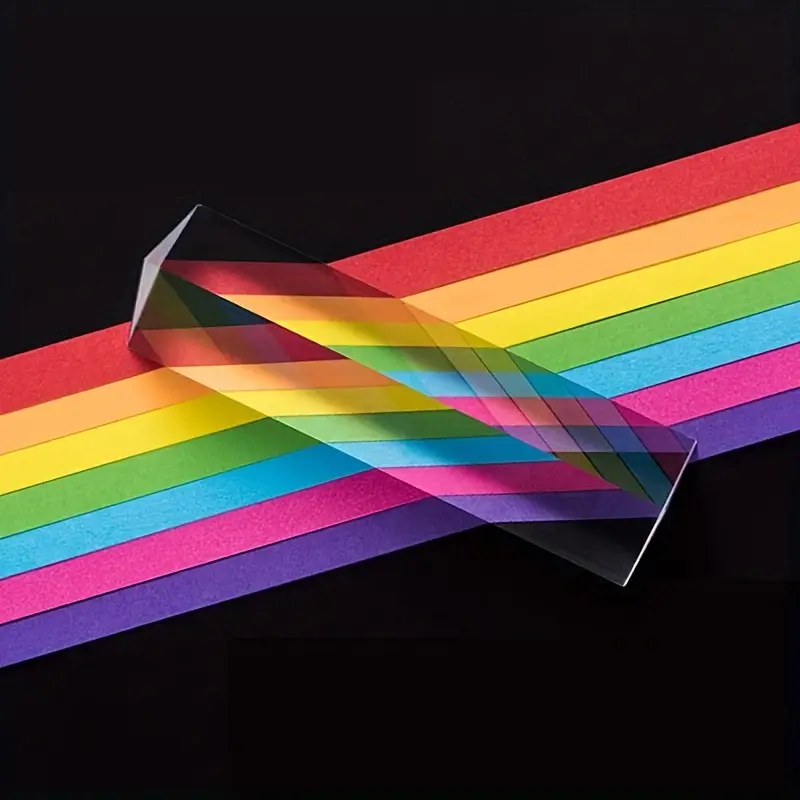The image features a bold, vibrant rainbow stripe set against a stark black background, running diagonally from the lower left to the upper right. The rainbow displays seven vivid colors: red, orange, yellow, green, blue, magenta pink, and purple, slightly differing from the traditional spectrum. Overlaying this dynamic stripe is a three-dimensional glass prism, shaped like a triangular post. The prism, although not the source of the rainbow, creatively distorts and reflects the array of colors beneath it, adding a chevron-like pattern at certain angles. The composition evokes a sense of joy and is reminiscent of the iconic Pink Floyd album art, albeit from a unique perspective.